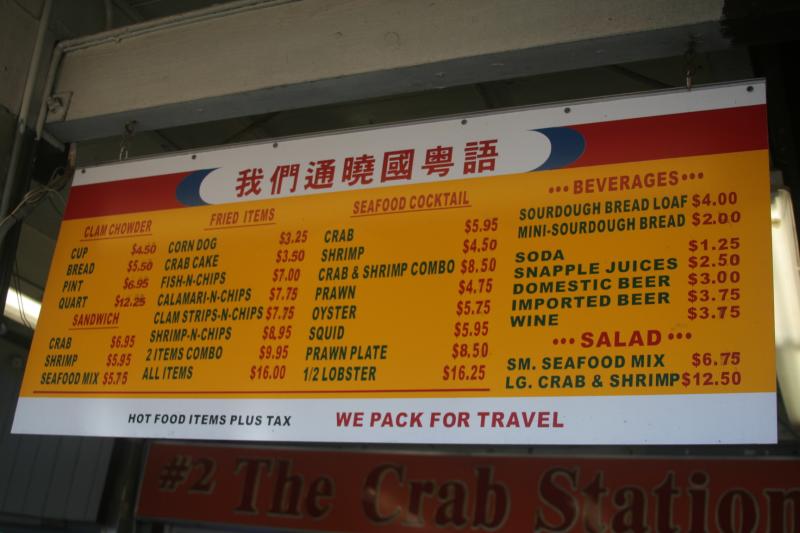This photograph captures a vividly colored menu hanging on a signboard from a metal post attached to the ceiling. The menu is richly detailed with colors predominantly in shades of red, blue, white, and gold, creating a striking visual appeal. The primary background color of the menu is gold, giving it a luxurious feel.

The menu items are categorized and listed as follows:

- **Clam Chowder (in red font)**
  - Cup: $4.50 (black font for "Cup", red font for the price)
  - Bread: $5.50
  - Pint: $6.95
  - Quart: $12.25

- **Sandwich (in red font)**
  - Crab: $6.95 (food item is in black, price in red)
  - Shrimp: $5.95
  - Seafood Mix: $5.75

- **Fried Items (in red font)**
  - Corn Dog: $3.25
  - Crab Cake: $3.50
  - Fish and Chips: $7.00
  - Curry and Chips: $7.75
  - Clam Strips and Chips: $7.75
  - Shrimp and Chips: $8.95
  - Two Items Combo: $9.95
  - All Items: $16.00

- **Seafood Cocktail (in red font)**
  - Crab: $5.95
  - Shrimp: $4.50
  - Crab and Shrimp Combo: $8.50
  - Prawn: $4.75
  - Oyster: $5.75
  - Squid: $5.95
  - Prawn Plate: $8.50
  - One Half Lobster: $16.25

- **Beverages (in red font)**
  - Sourdough Bread Loaf: $4.00
  - Mini Sourdough Bread: $2.00
  - Soda: $1.25
  - Snapple Juices: $2.50
  - Domestic Beer: $3.00
  - Imported Beer: $3.75
  - Wine: $3.75

- **Salad (in red font)**
  - Small Seafood Mix: $6.75
  - Large Crab and Shrimp: $12.50

At the bottom of the menu, it states in black font, "Hot Food Items Plus Tax." Additionally, in red font, it notes, "We Pack for Travel," indicating that all items are available for takeaway.